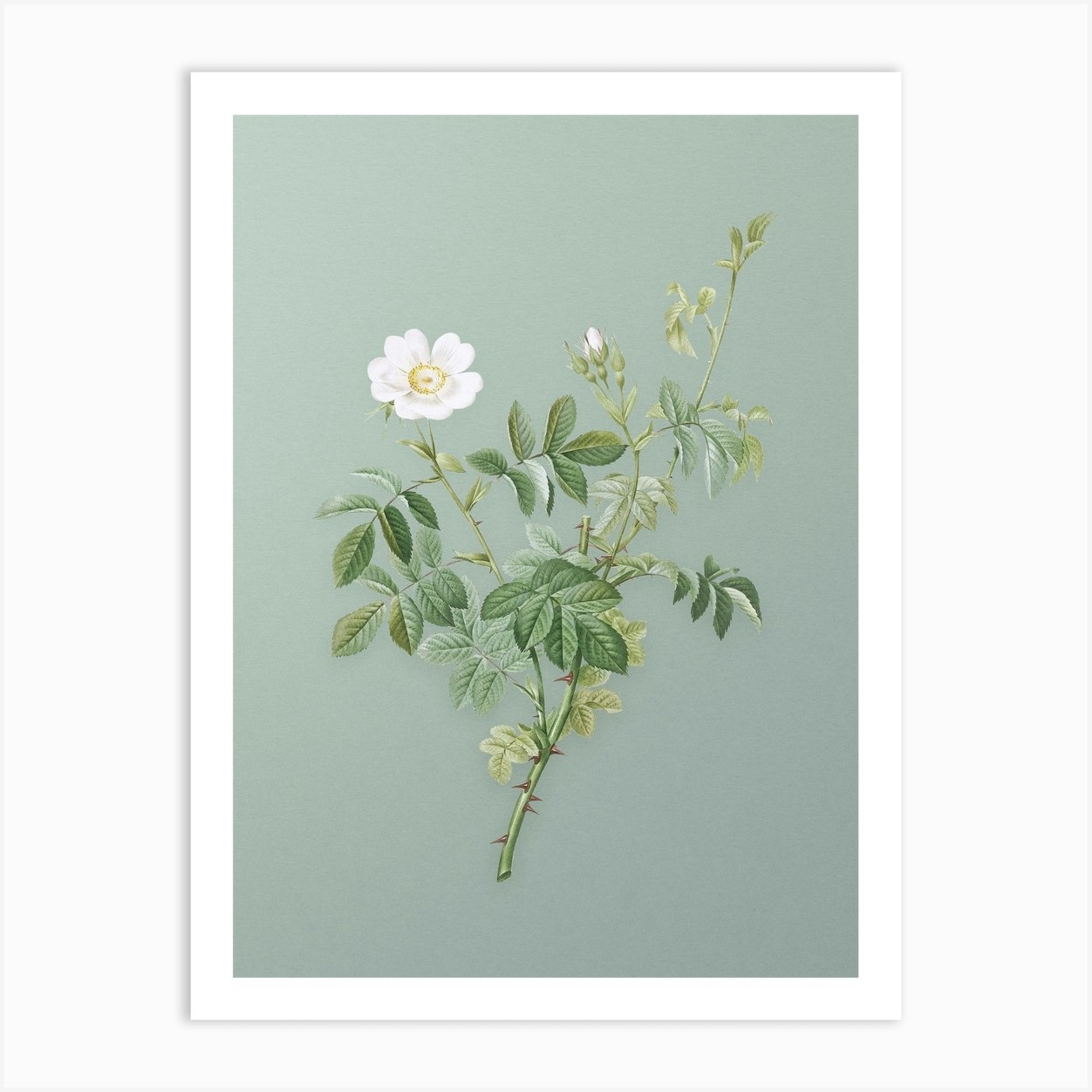The image features a detailed painting of a thorny green plant branch, set against a light gray to blue tinged background. The central focus is a beautiful white flower with five petals and a yellow center, situated on the upper left section of the artwork. Surrounding the flower are several buds on the brink of blooming and an abundance of green leaves interspersed with a few lighter-colored ones. The thorns are prominently visible at the lower part of the branch, which appears to have been freshly cut. The artwork is housed in a tall, vertical, white rectangular frame, adding a refined border to the composition.